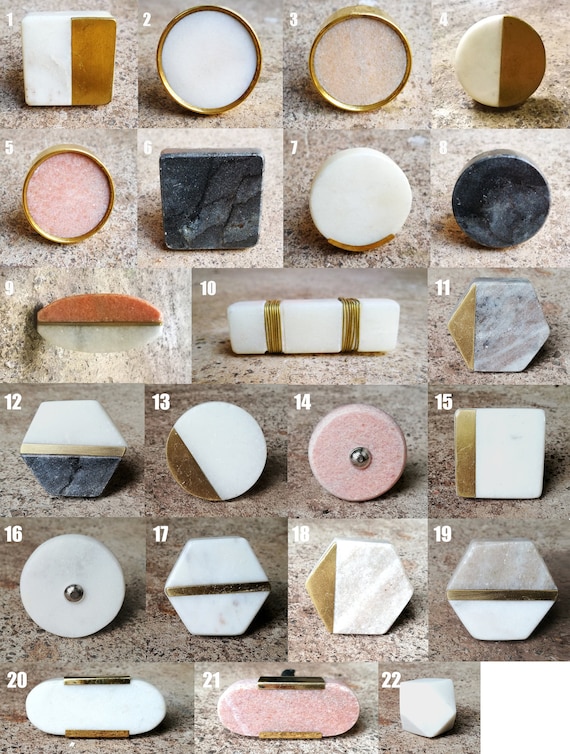The image features a collection of 22 distinct knobs or handles, each meticulously crafted from different types of stone and encased or accented with brass or gold. The display comprises various shapes such as hexagonal, octagonal, circular, rectangular, and square, and includes colors like browns, pinks, whites, grays, and blacks. Each item in the montage is uniquely numbered from 1 to 22, enhancing the clarity of the arrangement, which is set against a stone background and seemingly tilted up, suggesting a vertical display. Notable stone materials include marble and rose quartz, with some pieces incorporating black onyx. The emphasis is on the luxurious and diverse nature of the materials, unified under an elegant presentation that is likely intended for cabinetry hardware.